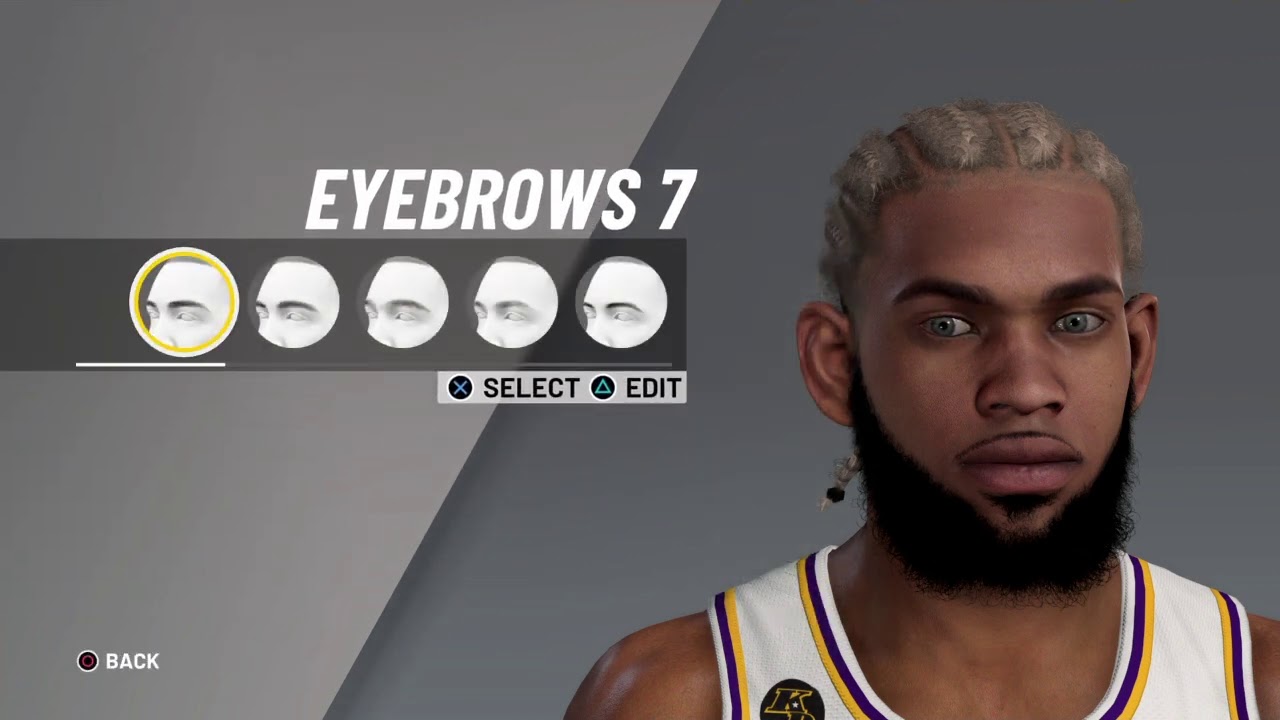A highly detailed and realistic in-game design screen showcases a basketball player with blonde cornrows and strikingly pale gray eyes. His defining features include a full black goatee and a white basketball jersey accented with purple and yellow stripes around the neck and armholes. The background is a gradient of dark to light gray, emphasizing the player's lifelike appearance. The user is in the process of customizing the player's eyebrows, as indicated by the large white text "Eyebrows 7" at the top of the screen. Below it, various eyebrow options are displayed, with the first option highlighted by a yellow circle. Additional interface elements include a yellow "X" for selecting, a triangle labeled "Edit," and a red "Back" button at the bottom left corner.